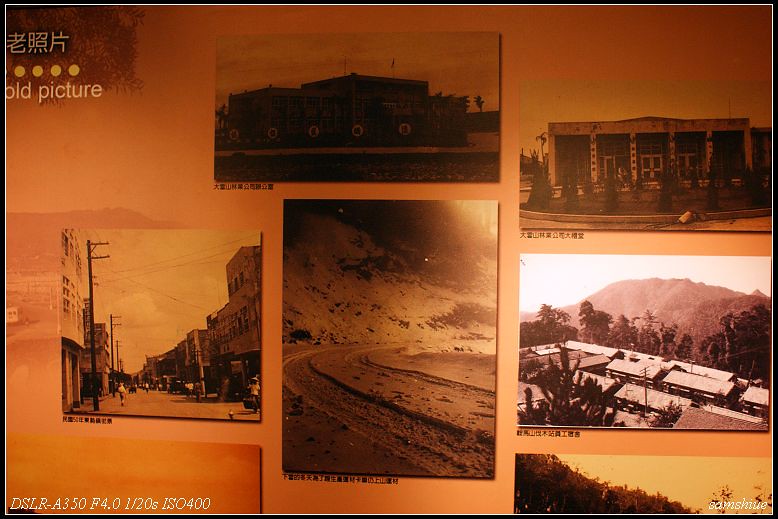This indoor photographic image showcases a series of black and white photos with an orange tinge, mounted on a wall. The central arrangement features five main photographs: four in landscape mode and one in portrait. The portrait photograph in the middle captures a serene beach scene. To its left, an old city street is depicted, while above it, a silhouetted wide building stands against the sky. On the right, a series of buildings with gabled roofs and a mountain in the background are visible, and above that, a single-story building with columns that appears to be a memorial or monument, with trees in the foreground. The image includes text with "OLD picture" and Asian characters at the top right, "DSLR-A350 F4.0 1-20S ISO 400" at the bottom left, and the word "SAMSHIUE" at the bottom right. Additional partial photos can be glimpsed at the bottom of the arrangement. The overall tone of the image is warm, dominated by an orange hue.